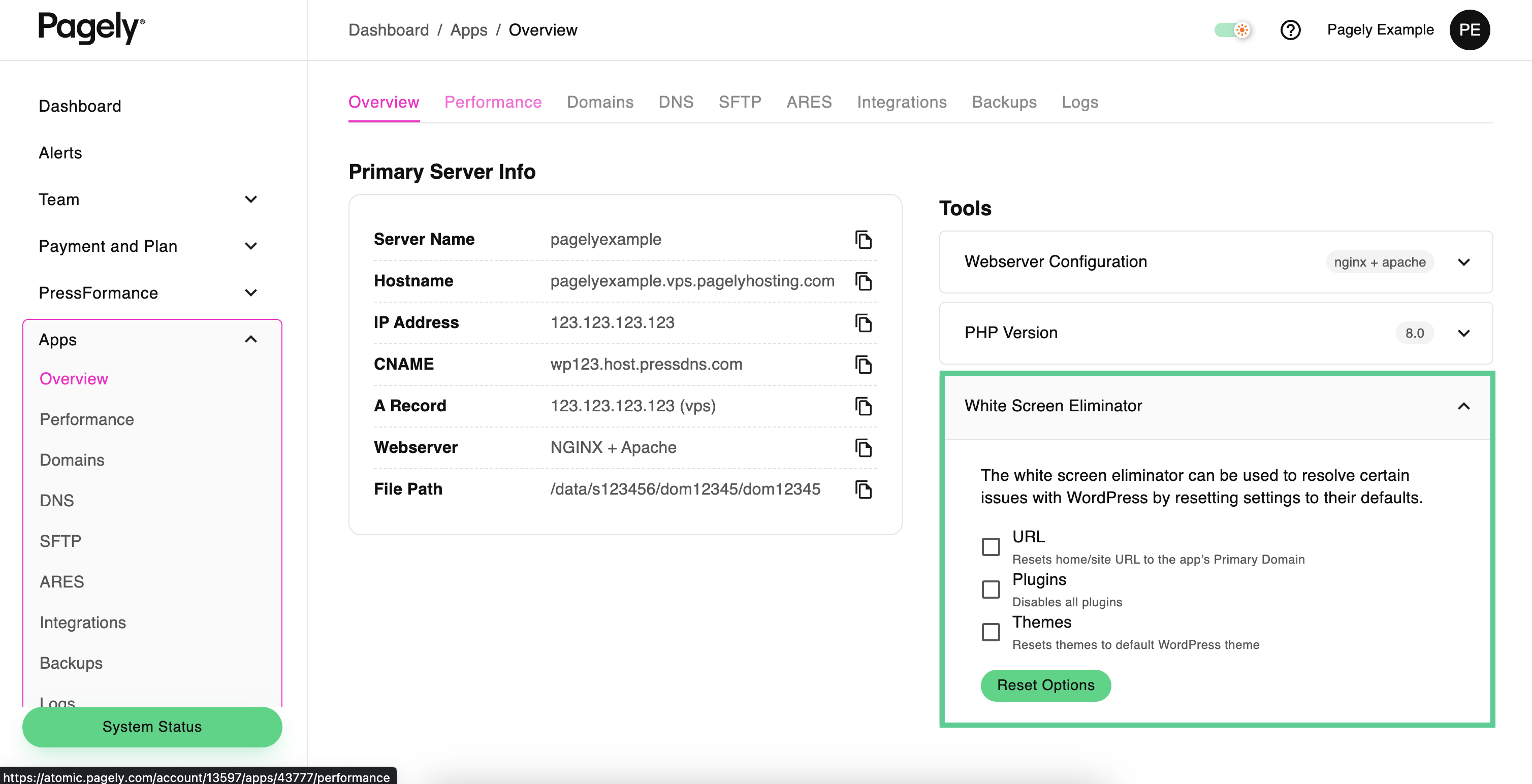The image showcases the main dashboard of a program called Pagely. This dashboard serves as a central hub, providing access to various features and functions. At the top right corner is a profile section, labeled as "Pagely Example," indicating it is a demonstration account. Accompanying the profile name is a circular black avatar displaying the initials "P" and "E."

Beneath the profile section, multiple categories such as "Private Server Info" and "Tools" are listed. These categories contain extensive information and options relevant to the user's needs. The interface is organized with different options highlighted in pink on the left side and green on the right side, allowing users to navigate between sections easily.

Several green bubbles, likely indicating actionable items or statuses, are visible throughout the interface. Towards the bottom of the dashboard, options for "System Status" and "Reset" are provided. The overall design of the page is predominantly white, with minimal use of color, lending it a clean and straightforward appearance.